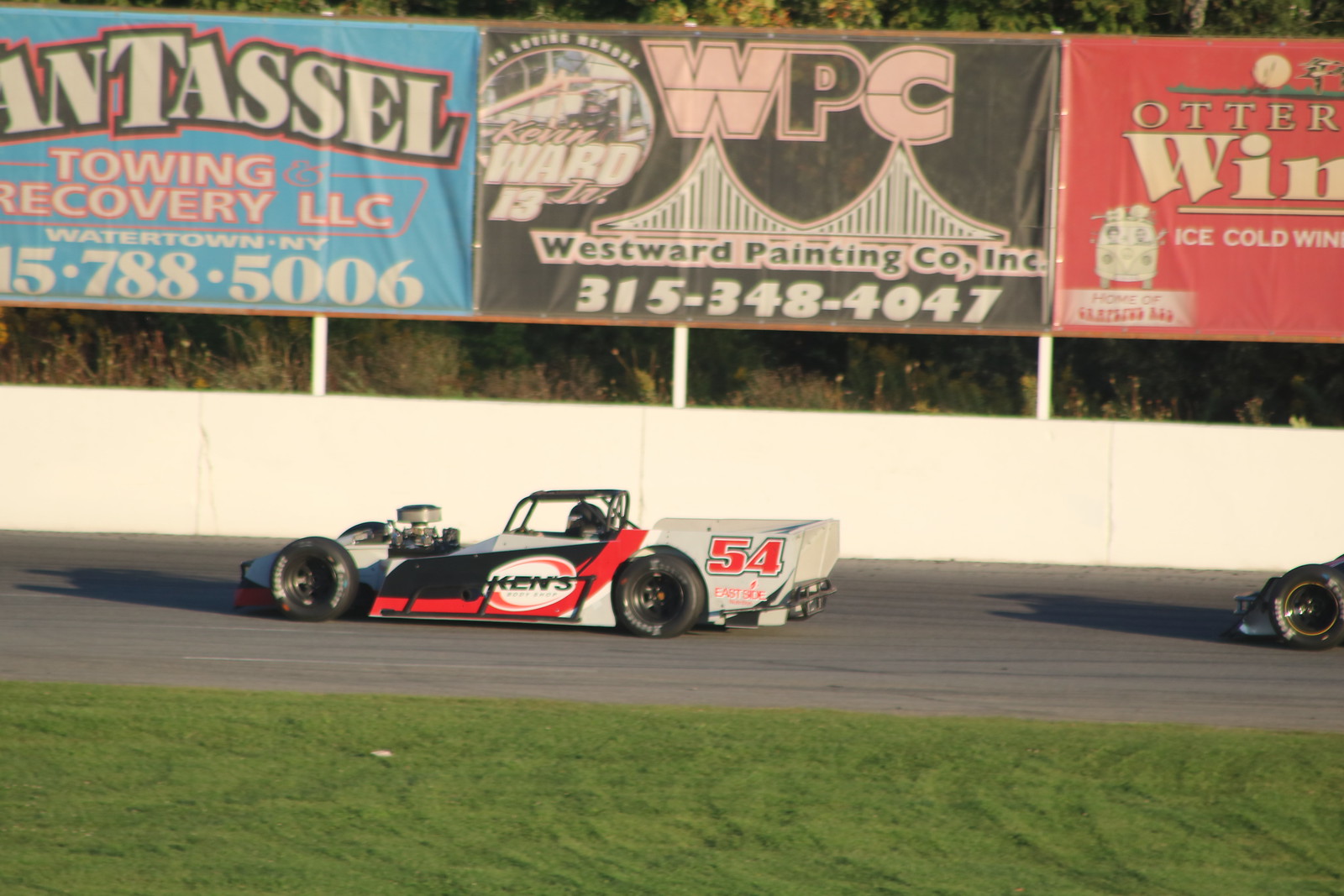The image portrays a thrilling moment on a professional racing track featuring open-wheel Formula One cars heading left. At the forefront is a striking car, predominantly grey, black, and red, with the number 54 emblazoned on its side. The sleek vehicle is notably low to the ground, with an exposed engine visible due to the absence of a hood, emphasizing its raw power. The driver, donning a black helmet, is encased in a black roll cage for safety. A notable sponsor, "Ken's," is displayed in white lettering inside an oblong circle with red swirled accents around its top and bottom edges.

Behind the primary car, a glimpse of another black car is visible, though most of it is out of frame. The scene is set during what appears to be either dusk or dawn, suggested by the long shadows stretching across the track. The background features a white retaining wall adorned with various posters, including a blue one partially reading "ANTASSE" and advertising a towing recovery service, a black poster with white and pink text “WPC” for Westward Painting Company, and a red one that ambiguously mentions “otters” and “ice cold wind.” Below the wall lies a patch of green grass, adding a touch of nature to the high-speed drama.